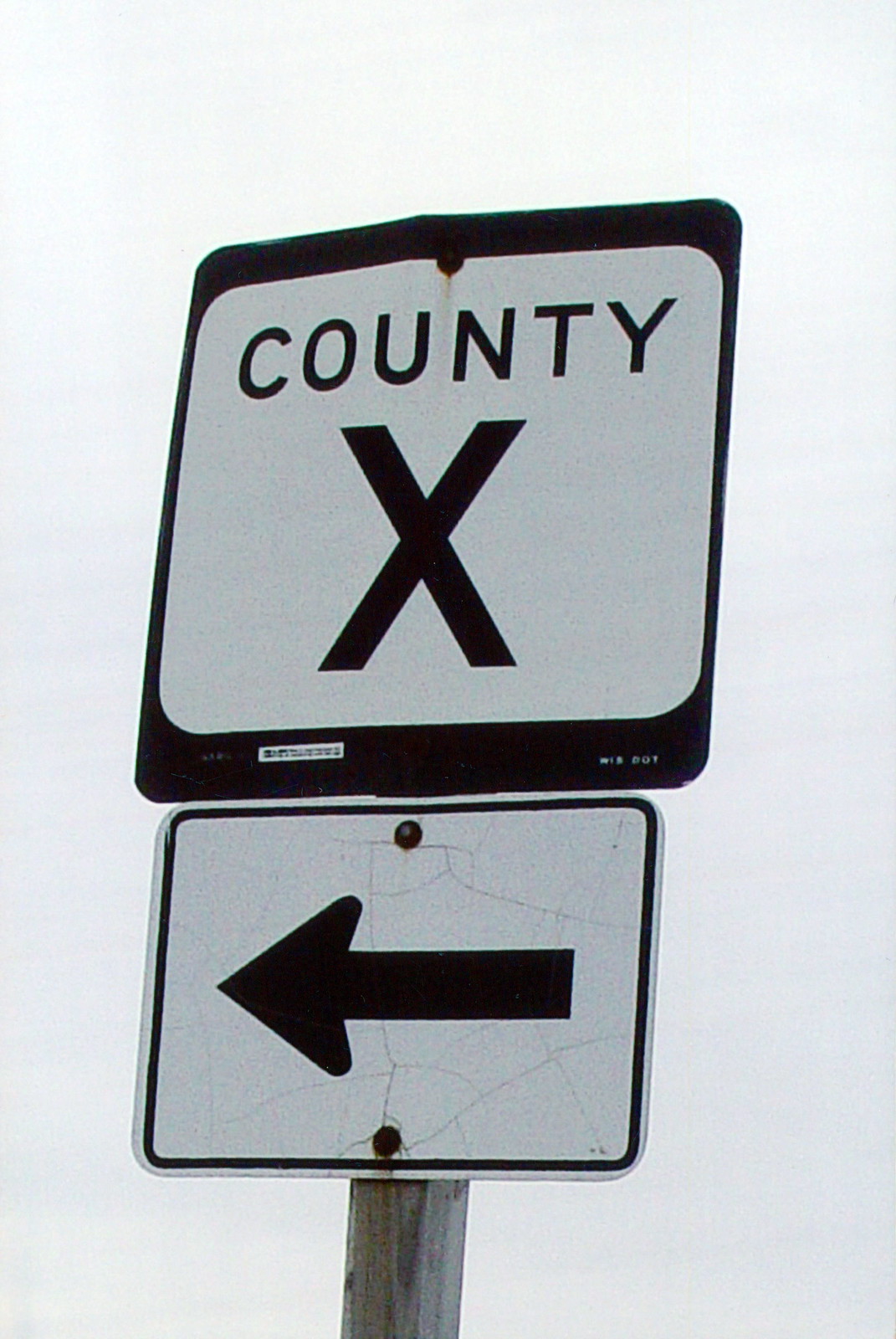In this simplistic yet striking image, the background features a serene, light blue sky, creating a tranquil atmosphere. Set against this calm backdrop is a wooden pole with two distinct signs mounted on it. The lower sign, secured with two bolts, has a minimalist design: a white background framed by a thin black border and marked with a bold black arrow pointing left. Above this directional sign is a larger, more square-shaped sign with a thicker black border. The word "COUNTY" is prominently displayed in black letters against the white background. The most eye-catching element, however, is the enormous black X that dominates the entire upper sign, becoming the focal point of the image and irresistibly drawing the viewer's gaze. This simple yet powerful composition effectively captures the viewer's attention, making the large X the central element of the scene.